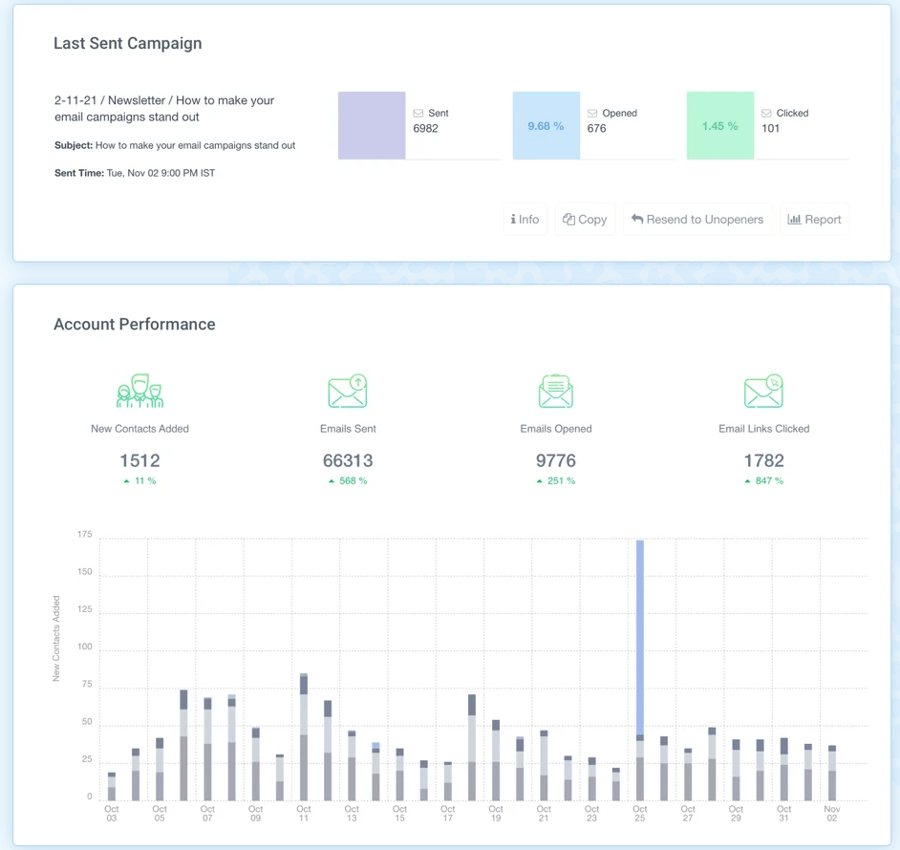The image displays a detailed view of an email campaign report in spreadsheet or software format. The top section of the page features a header against a white background, highlighted with a blue strip. Key information is listed from left to right:

- **Last Sent Campaign:** "2-1121 Newsletter"
- **Campaign Subject:** "How to Make Your Email Campaign Stand Out"
- **Time Sent:** Tuesday, November 2nd, 9:00 PM Eastern Standard Time

Beneath this header, there are three colored boxes that summarize the campaign performance metrics:
- **Lilac Box (Sent):** 6,982 emails sent
- **Blue Box (Opened):** 9.68%, which amounts to 976 opened emails
- **Green Box (Clicked):** 1.45%, equaling 101 clicks

Further below, the section titled "Account Performance" presents a graph depicting varying levels of activity. The performance statistics detailed from left to right are:
- **New Contacts Added:** 1,512 (11% increase)
- **Emails Sent:** 66,313
- **Emails Opened:** 9,776
- **Email Links Clicked:** 1,782

This comprehensive visual provides critical insights into the reach and engagement of the email campaign.